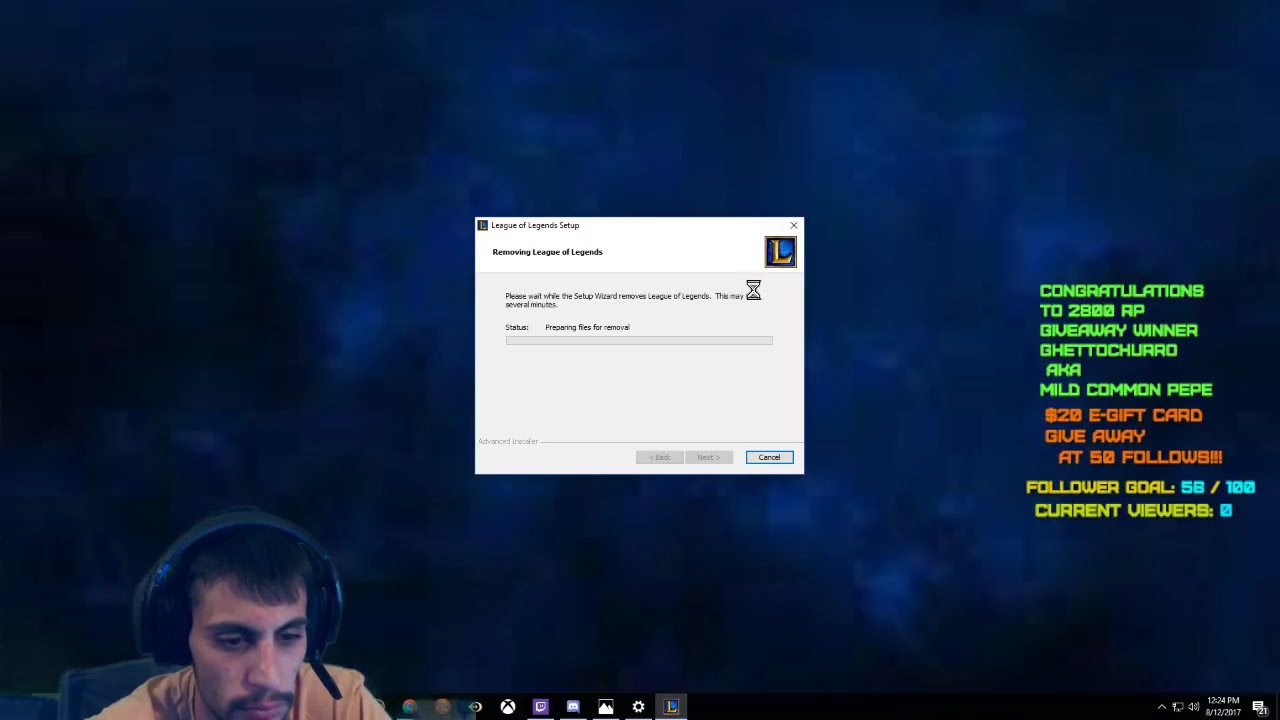The image depicts a Windows desktop screen with a swirling dark blue and black cloud-like background. In the center, a white pop-up window for the League of Legends setup is prominently displayed, indicating that the software installation is in progress with an hourglass icon and buttons including "Cancel." To the right of this pop-up, vibrant text in various colors conveys several notifications: in green, "CONGRATULATIONS TO 2800 RP GIVEAWAY WINNER GHETTO CHURRO AKA MILD COMMON PEE-PEE," followed by an orange announcement, "$20 E-GIFT CARD GIVEAWAY AT 50 FOLLOWS," and in yellow, "FOLLOWER GOAL 58 OUT OF 100, CURRENT VIEWS: 0." At the bottom left corner, a reflection of a man wearing over-the-ear headphones and sitting in front of the computer is visible; he appears to be attentively engaged with the screen. The Windows taskbar runs along the bottom, affirming the desktop environment.